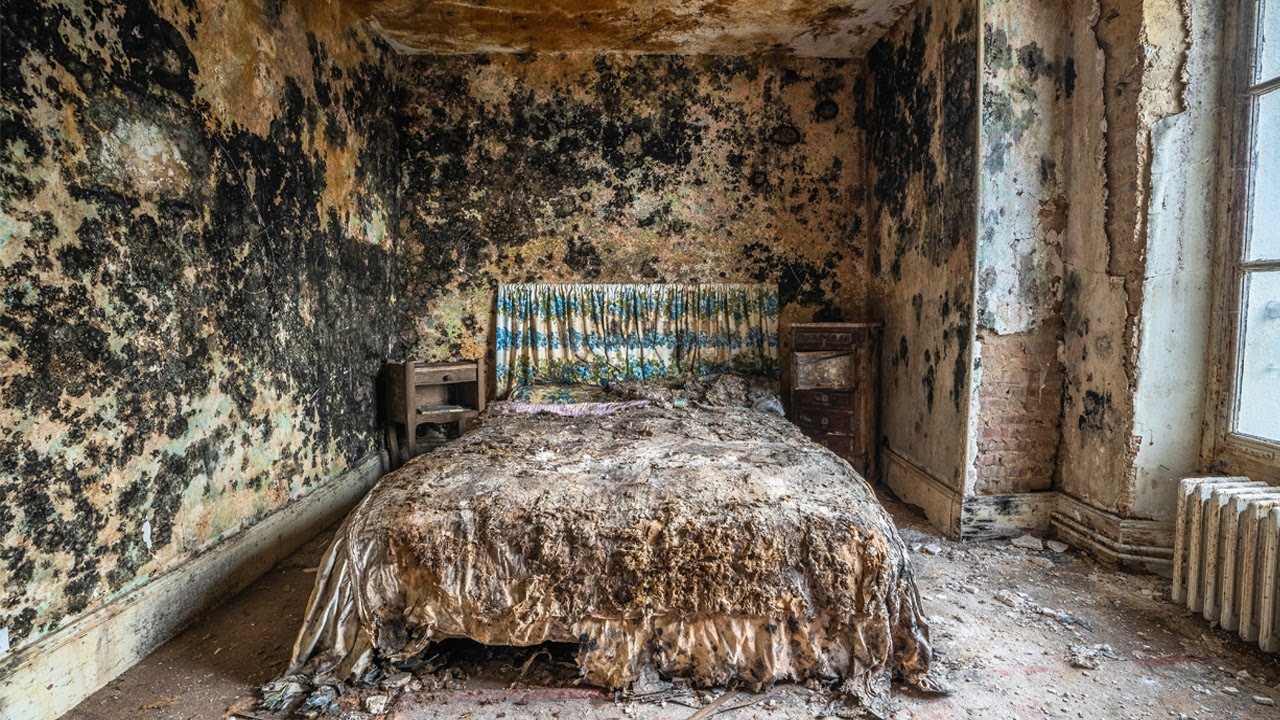The image depicts a highly deteriorated and dilapidated bedroom, evoking a sense of decay and abandonment. The focal point is a double bed situated in the center, viewed from the foot. The bed is covered with a dirty, torn comforter that was once colorful but now shows patches of light brown, white, and various worn colors. Beneath the comforter, an orange, tattered bedsheet is partially hanging out. Draped over the headboard is a piece of cloth that still retains some light blue, white, and rusty orange hues, adding the only semblance of color to the otherwise bleak room.

The walls, visible on three sides—left, right, and back—are heavily deteriorated, marked with black and rust-colored spots, and pockmarked by mold. The paint is cracked and peeling, exposing the bricks behind in several areas. The floor, grimy and covered with debris and small pieces of deteriorated fabric, lacks any carpeting. Alongside the bed, there are small, wooden nightstands on both sides, contributing to the room's cluttered appearance.

On the right side of the image, a partially visible white radiator sits beneath a tall window, which is mostly cut off from view. The window appears to have three panes, allowing light to spill into the otherwise dim room. Despite the room's poor condition, the photograph is clear, high-quality, and well-lit, capturing the full extent of its decay and evoking a post-apocalyptic atmosphere.